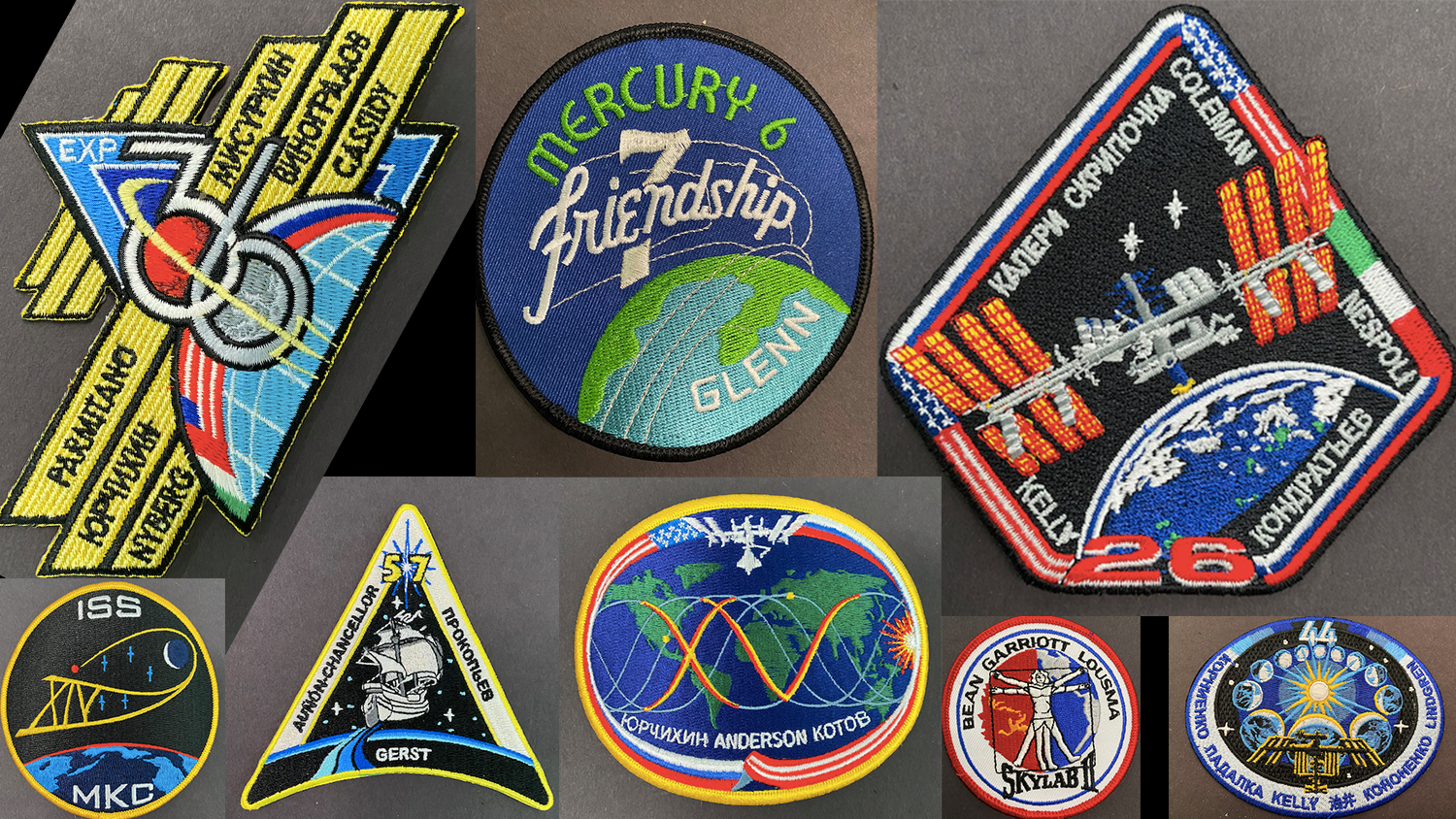The image displays a collection of eight space-related patches, each signifying different missions and international cooperation. The top left patch, featuring the text "EXP-76" along with six names, has a stylized design incorporating both the U.S. and Russian flags over a view of Earth, indicating a multinational mission, possibly related to the International Space Station (ISS). The next patch prominently reads "Mercury 6 Friendship 7" and includes the name "Glenn," alongside imagery of Earth in green, blue, and white hues. Another triangular patch, with names "Kelly," "Kondratiev," and "Coleman," features text in Russian, and displays flags of the US, Italy, and Russia, suggesting it represents a collaborative ISS mission, marked with the number "26." 

In the bottom left, a simpler patch tags "ISS-MKC," potentially another ISS-related emblem. Adjacent is a patch marked "57" and adorned with the name "Gerst," likely commemorating Alexander Gerst's mission. Among the patches, one carries a stylized sailing ship set against a space backdrop. There is also an anatomical illustration patch with "Skylab 2," credited to Bean, Garriott, and Luzma. Concluding the collection, the final patch shows multiple globes encircling the Sun with a satellite foreground, numbered "44." These patches collectively celebrate various NASA missions and the spirit of international space camaraderie.